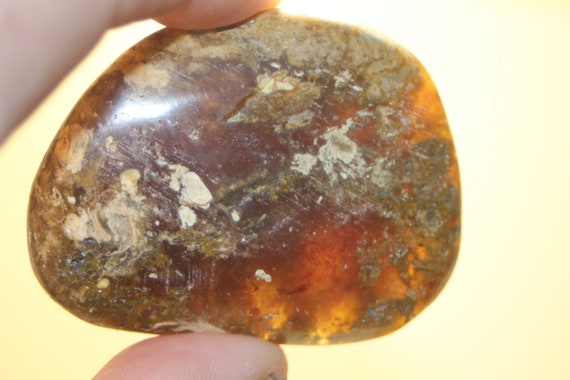This image features a detailed close-up of an oblong, amber-colored stone being held by the cropped tips of a left hand's thumb and index finger against a soft butter-yellow background that is backlit with a bright orange glow. The stone, which dominates the frame, measures a couple of inches tall by a few inches wide and has a smooth surface free of rough textures. While primarily amber, the stone showcases a variety of hues and textures: patches of white, tan, gray, and more opaque brown areas intermix within its matrix. Certain areas towards the right side of the stone appear semi-translucent, allowing light to shine through and create glowing edges, while a hot highlight in the upper left corner suggests light reflection. Despite some scuff or cut marks hinting at its extraction, the stone remains largely smooth, with variations in thickness visible through the light's play on its surface.